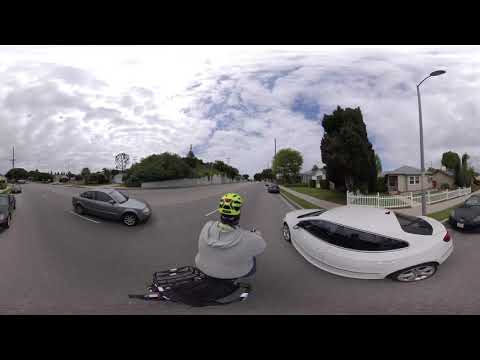In this fisheye photo of a quiet suburban neighborhood, a large man on a moped dominates the foreground, dressed in a gray sweatshirt and a green safety helmet. Amidst the distorted perspective, he maneuvers between a small white sedan with tinted windows and chrome wheels on his right and a gray sedan on his left. The road beneath them is gray asphalt adorned with dotted white lines. To the right, a house with a white picket fence stands next to a light pole, while the left side of the frame features a cluster of green trees. Further ahead, another car is parked on the right side of the street. The sky above is mostly cloudy, with patches of blue peeking through, casting a subdued light on the scene. The entire image has a bowed, panoramic feel, distorting the spatial relationships between the objects and making the neighborhood look more surreal and compact.